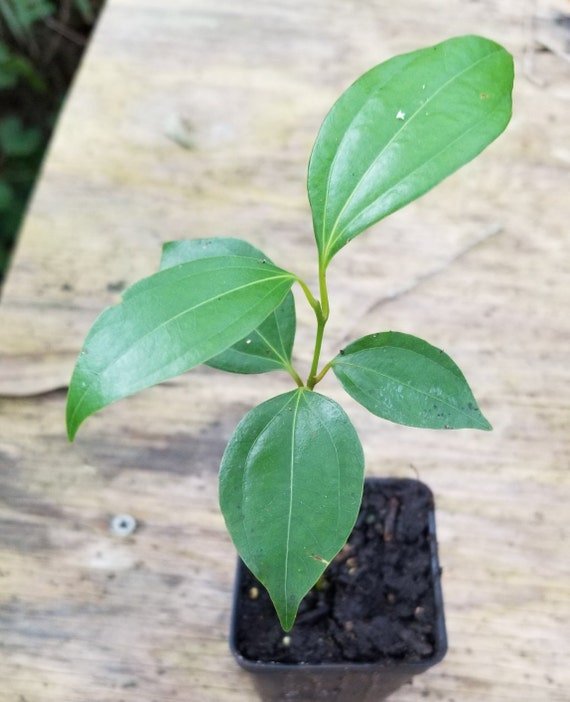The image is a vertically aligned rectangular close-up of a small plant in a black, square-shaped plastic container, typical of those purchased from a nursery. The container is filled with rich, black soil, dotted with tiny brown speckles. The plant features a single thin green stem with five large, rounded green leaves extending in different directions: one towards the upper right, one to the right, one to the upper left, one to the left, and one pointing downwards. The background consists of a light brown wooden surface, which is weathered and adorned with dark stains and a silver screw drilled into it. The photo captures an outdoor scene with blurry greenery visible in the upper left corner, suggesting more plants or branches lying on the ground below the table on which this highlighted plant sits. Overall, the plant appears healthy despite lacking blooms, and its solitary container hints it may soon be transplanted.